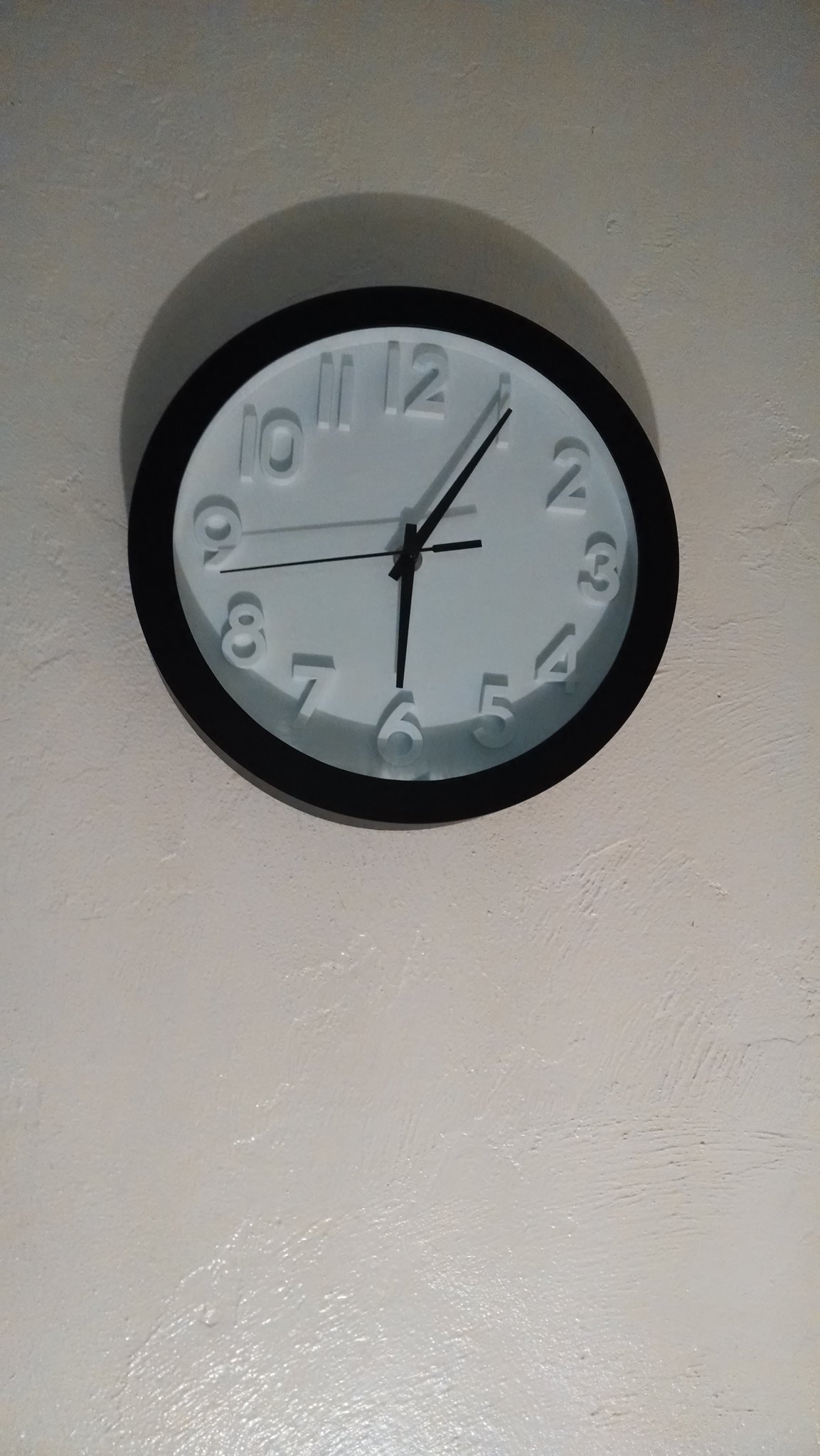A sleek clock is mounted on a white, glossy wall adorned with a subtle, swirling pattern. The clock features a thick black frame, contrasting sharply with its white face. It has bold black hour and minute hands, coupled with a slim black second hand. The numerals are also white but are raised, giving them a three-dimensional appearance against the otherwise flat face of the clock. Positioned near the center top of the image, the photograph appears to be taken from a low angle, looking upward. A semicircular shadow above the clock suggests that the light source is either from below or that a camera flash was used, adding an interesting highlight to the scene.